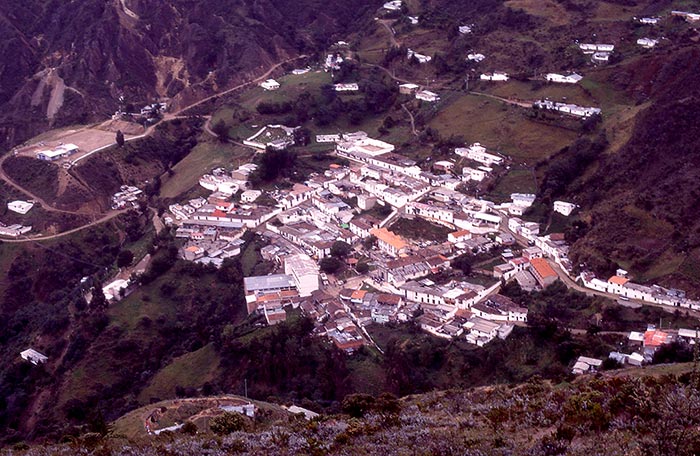This stunning aerial photograph captures a picturesque small town nestled on a lush, green hillside. The image, possibly taken from an airplane, helicopter, or drone, offers a high-altitude perspective showcasing the town’s landscape features prominently. The town is characterized by predominantly white buildings with vibrant red roofs, clustered closely together in the center and becoming more sparsely distributed as they extend towards the mountainous background. 

The surrounding countryside is rich with green hills and flatlands, interspersed with occasional rocky and brownish mountainous features. Narrow, likely dirt roads weave through the town, connecting the central cluster of buildings with more isolated structures on the outskirts. The lower portion of the image, primarily to the left, depicts a mix of green vegetation and scattered trees, though the area appears less densely populated with trees and absent of visible people or vehicles. The overall scene is a harmonious blend of well-arranged homes and natural landscapes, painting a serene and orderly rural setting.